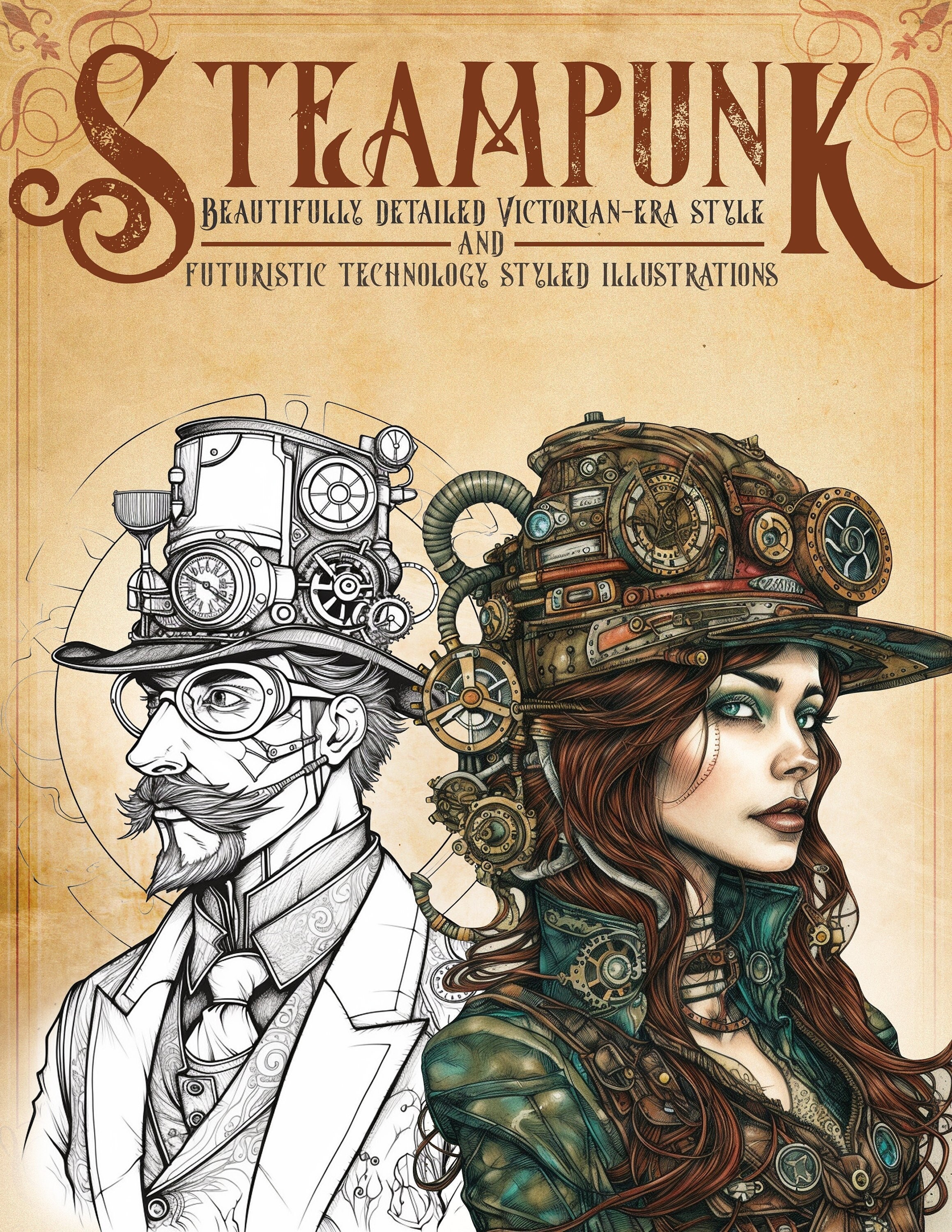The cover of the book or magazine features a prominent title "STEAMPUNK" in large red capital letters with a striking interplay of letter sizes, where the S and K are slightly elongated. Below the title, in black text, the phrases "Beautifully Detailed Victorian Era Style" and "Futuristic Technology Styled Illustrations" are neatly laid out, separated by a red horizontal line at the word "and."

On the left side, there's a detailed black and white illustration of a man. He is facing slightly forward and to the left, adorned with a tall hat embellished with various gears and machines. He sports glasses, a thin pencil mustache, and a beard, complementing his white suit and tie.

To the right, a vividly colored drawing of a woman contrasts the man's monochromatic appearance. She faces slightly forward and to the right, wearing a brown hat similarly decked out with multi-colored gears and mechanical elements. Geometric details also adorn her jacket and collar. Her long red hair cascades in front of her chest on both sides.

The cover merges the elegance of the Victorian Era with the inventive spirit of futuristic steampunk technology through its intricate illustrations and thoughtfully crafted text.